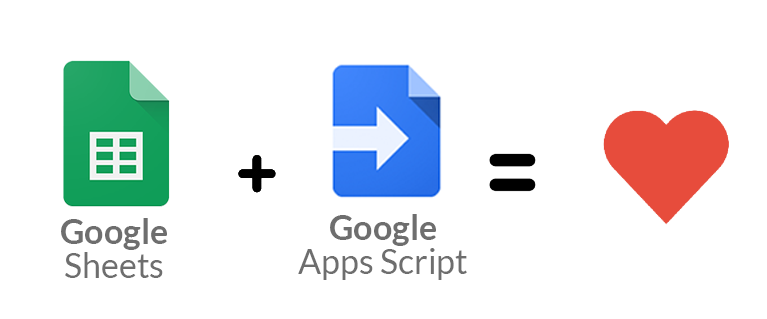The image features a symbolic equation on a completely white background. On the left side, there is a green icon representing Google Sheets, which has a folded corner and a white window with rows and columns. Below this icon, the text "Google Sheets" is written. To its right, there is a black plus sign followed by a blue icon symbolizing Google Apps Script. This blue icon also has a folded corner with a white arrow pointing right, and the text "Google Apps Script" is written below it. Adjacent to this is a black equals sign, leading to a red heart symbol. Overall, the image conveys the message that "Google Sheets plus Google Apps Script equals love," suggesting that these tools work well together.